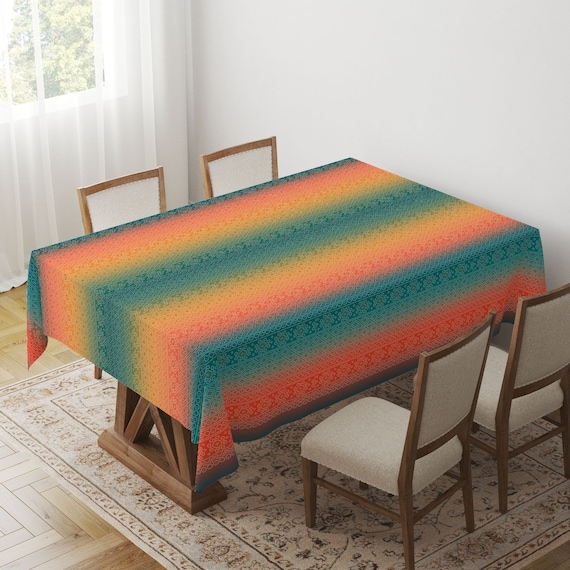The photograph depicts a dining area with a central large rectangular wooden table placed against a white-painted wall. The table stands on a brown checkered hardwood floor and is partially covered by a tan and brown area rug featuring various irregular designs. Positioned under the table are four wooden chairs, each with white seat cushions and backs. The table's leg and frame, made of brown wood, are visible beneath the multicolored tablecloth that drapes over it with a repeating pattern of dark blue, pink or red, teal, yellow, and green stripes.

Behind the table, the adjacent white wall features a window outlined by a white frame filled with glass panels, mostly obscured by sheer, semi-translucent curtains. The overall shape of the photograph is square, with equal lengths on each side, emphasizing the symmetrical layout of the room. The photo captures a cozy dining setting, accented by the vibrant hues of the tablecloth and the elegant simplicity of the wooden furniture and flooring.